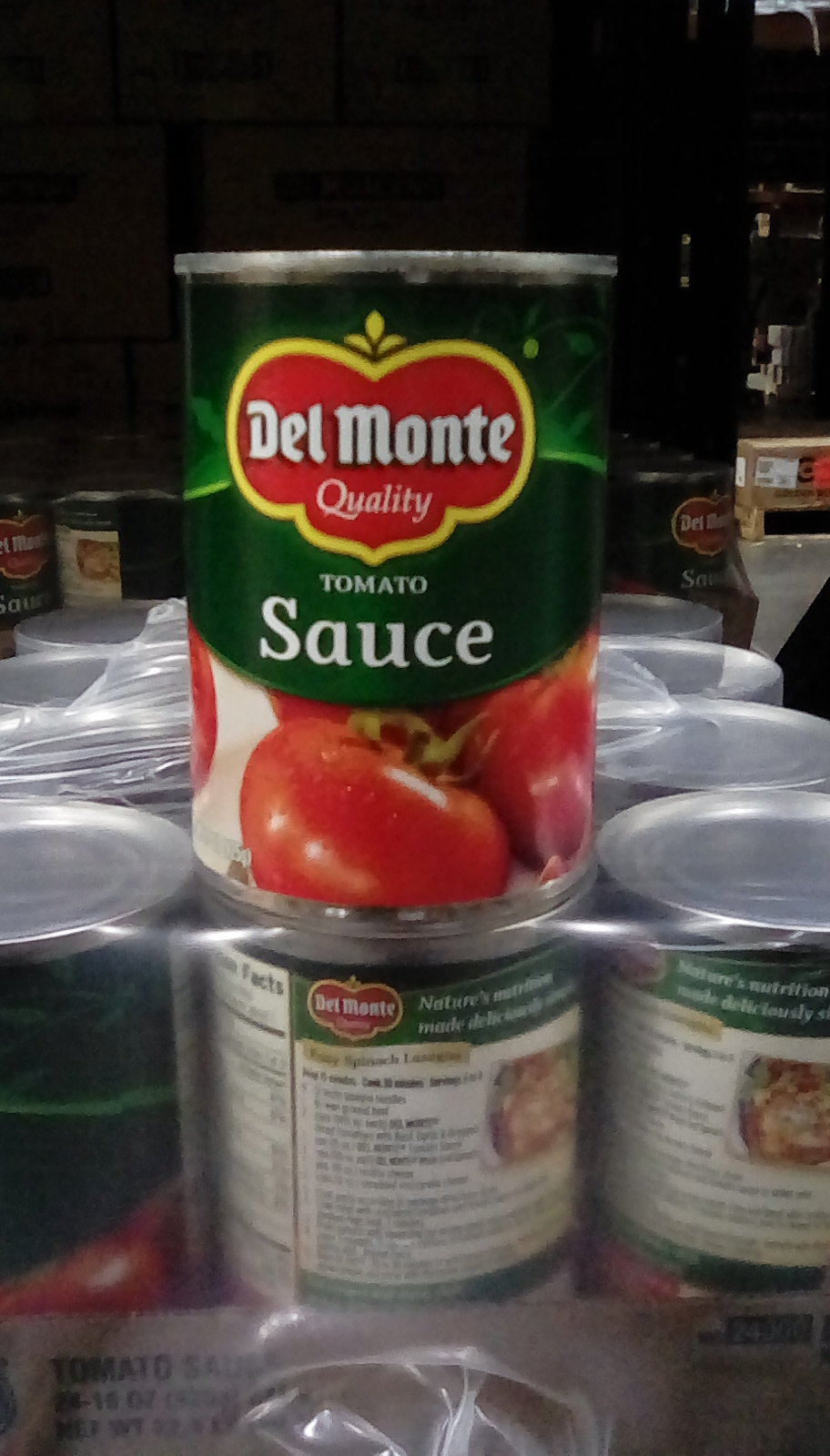This color photograph features an organized display of Del Monte tomato sauce cans. At the forefront, a single aluminum can prominently sits, unwrapped, atop a shrink-wrapped palette containing multiple identical cans. The can itself is detailed with a hunter green label that prominently features the Del Monte quality logo, a red heart-shaped icon outlined in yellow. Directly beneath this logo, the words "tomato sauce" are emblazoned in white font against a green background, and a vivid photograph of ripe red tomatoes is displayed on a white section of the label. The can has a silver top and bottom and is circular in shape. This unwrapped can appears to have been removed from the left front portion of the case below, which is housed in a brown box marked with the inscription "tomato sauce" on its side. In the background, the shrink-wrapped case contains at least twelve cans in the top row, their labels facing backwards, revealing another Del Monte logo and a recipe, though the text is too small to read. The photograph is vertical in orientation and does not include any people or animals.